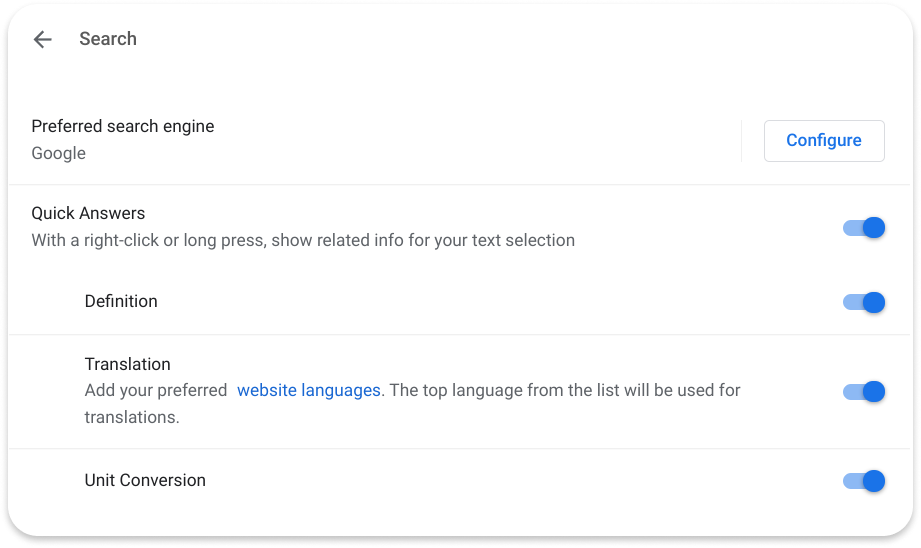**Detailed Caption:**

The image is a detailed screenshot of the configuration and settings page of a search engine. The screenshot itself is rectangular, with the top and bottom sides being significantly longer than the left and right sides. The corners of the rectangle within the screenshot are rounded, and a light gray border surrounds the central white rectangle. Outside this central rectangle, the border area is solid white.

At the top left corner of this central rectangle, a black arrow points towards the left and is accompanied by the text "Search." Directly below this, the text reads "Preferred Search Engine, Google," indicating the default search engine setting. To the right of this line, there is a small white rectangle with a gray border containing the text "Configure."

A gray line runs horizontally from left to right, separating the top section from the rest of the settings. Below this, the text "Quick Answers with a right click or long press show related info for your text selection" appears, with a blue toggle switch on the far right side that is currently turned on.

Further down, the text "Definition" is aligned to the left, accompanied by another toggle switch on the right side, which is also turned on. Below this, the setting "Translation, add your preferred website languages. The top language from the list will be used for translations" is listed, with an activated toggle switch on its right.

Finally, at the very bottom, there is the "Unit Conversion" setting with yet another toggle switch on the right, which is turned on as well. This detailed configuration screen provides various toggles to customize the search engine's additional functionalities.